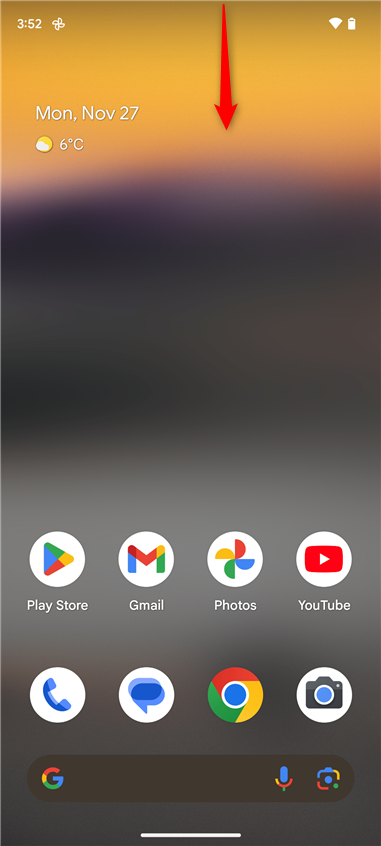The image is a vertically-oriented mobile screenshot showcasing various on-screen elements. In the top left corner, the time is displayed as 3:52, while the top right corner shows a nearly fully charged battery icon with a quarter circle next to it, indicating additional status information. Prominently featured is a red downward arrow originating from the top edge of the screen. 

The indistinct background features a gradient blur starting with an orange hue at the top, transitioning to purples, then darkening to black, followed by lighter to darker shades of gray as it descends towards the bottom.

In the top left section, the date is displayed in white text as "Monday, November 27." Below the date, it reads "6°C" accompanied by an icon depicting a yellow sun partially hidden by a white cloud, suggesting the current weather condition.

Dominating the bottom half of the screenshot are two rows of app icons arranged in a grid of eight circles, with four icons per row. The top row consists of the Play Store, Gmail, Photos, and YouTube icons. The bottom row features icons for a blue telephone, a blue speech bubble, the Google Chrome logo, and a camera. At the very bottom, there's a Google search bar ready for input.